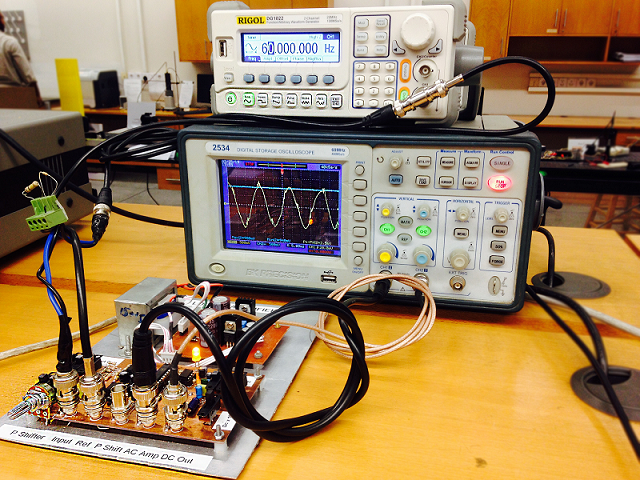The image depicts an electronics laboratory setting with a focus on a research-grade apparatus. Centrally, there's a rectangular machine resembling an oscilloscope, featuring a small monitor displaying yellow zigzag lines, indicative of waveform readings. The machine is adorned with an array of buttons, both grey and variously lit in green, yellow, and red. Below, a mess of wires connects to a motherboard with multiple shiny, screw-like connectors. At the top, a secondary device marked "60,000 Hz" or "60 million Hertz" has its own set of smaller buttons. All this equipment is positioned on a bright yellow-stained, wooden table. Behind it, other lab furniture like cabinets and tables are visible, suggesting this scene takes place in an educational or training center for electrical studies.